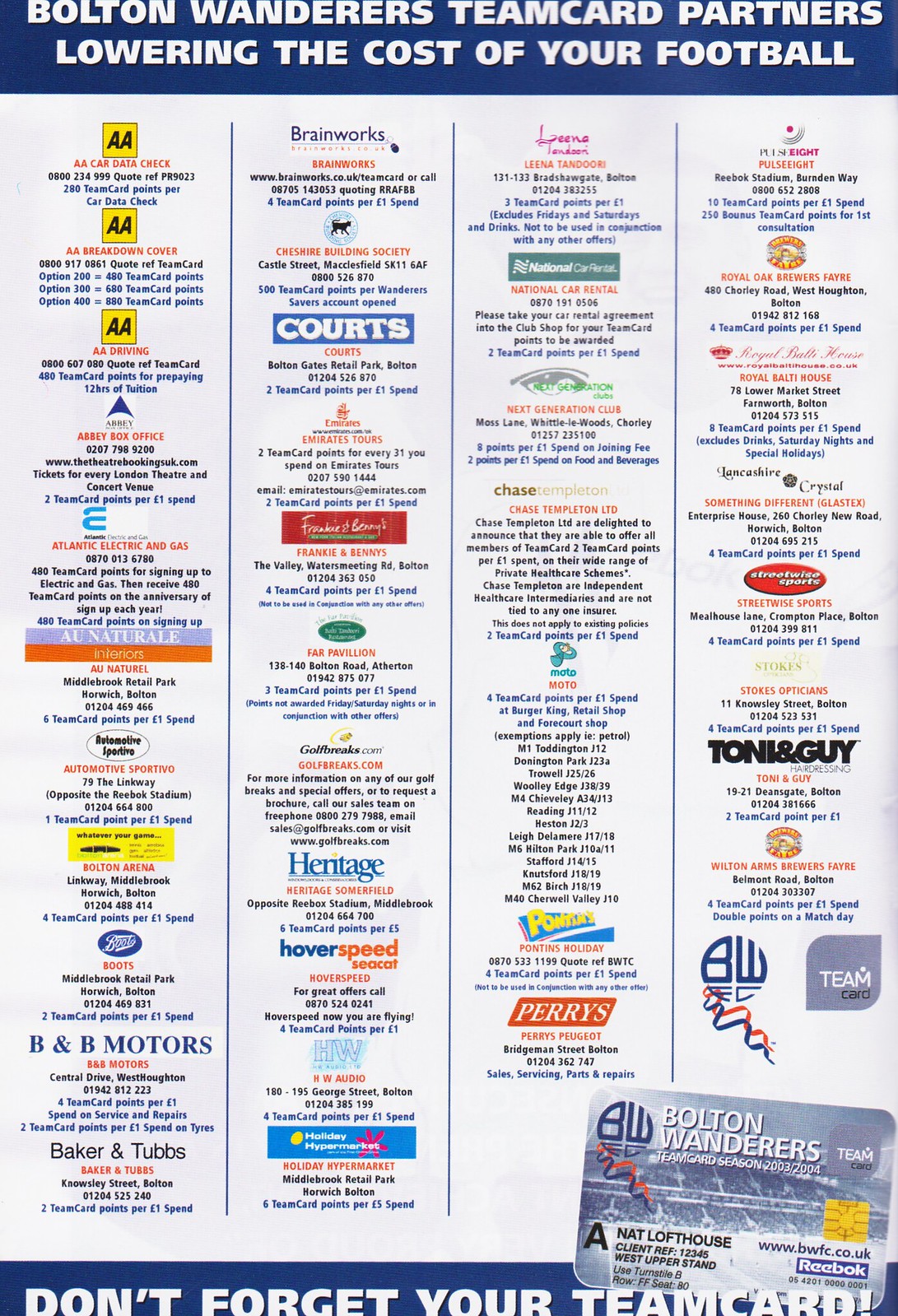The graphic titled "Bolton Wanderers Team Card Partners, Lowering the Cost of Your Football," features a predominantly white background accented by colorful prints and banners. At the top, a blue banner with white capital letters reads, "Bolton Wanderers Team Card Partners, Lowering the Cost of Your Football." The graphic is divided into four columns, each separated by a thin blue line, listing various businesses that support the Bolton Wanderers football. These columns include names of sponsors like B&B Motors, Baker and Tubbs in the first column, Quartz, Brainworks, and Hentage in the second, and Perry's and Tony and Guy in subsequent columns. Each ad is vibrantly colored in shades of purple, red, blue, and orange. At the bottom, another blue banner reminds readers, "Don't Forget Your Team Card." Alongside this, in the bottom right corner, there's an image of the Bolton Wanderers Team Card, designed to resemble a silver credit or bank card with white lettering.